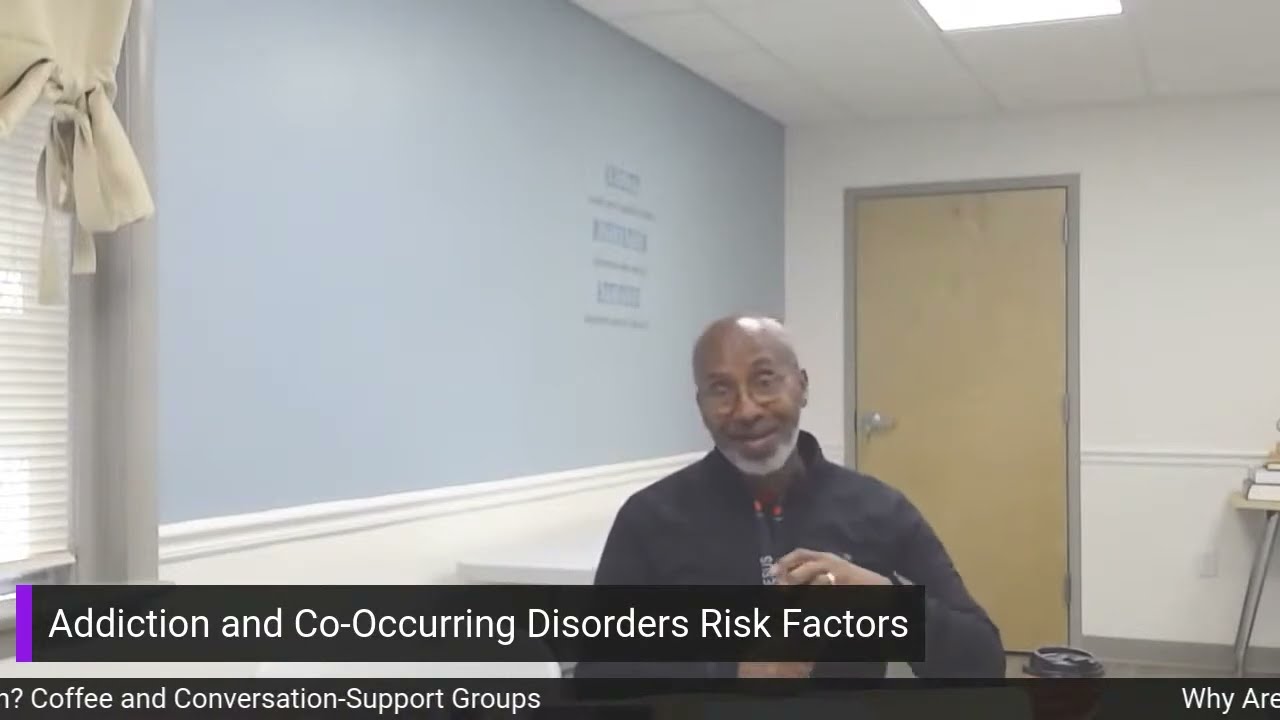This image, potentially a still from a video or a live stream, features an older black man, who appears to be in his 50s, with a bald head and a white beard. He has dark brown skin, circular glasses, and is wearing a black zip-up sweatshirt along with a black lanyard. The man is looking forward with his mouth partially open, possibly smiling or mid-speech.

He is seated in a room with a light powder blue wall behind him and a wooden door with a gray frame to his right. The door appears closed, and there is a fluorescent light shining from the white-tiled ceiling above. To the left in the room, there's a white wall with a window that has a gray border and closed blinds.

At the bottom left of the image, there is a black caption box with white text that reads, "Addiction and Co-occurring Disorders Risk Factors." Below that, the text continues to say, "Coffee and Conversation Support Groups." In the lower right corner, there is partial text starting with "Why are," but the rest is cut off.